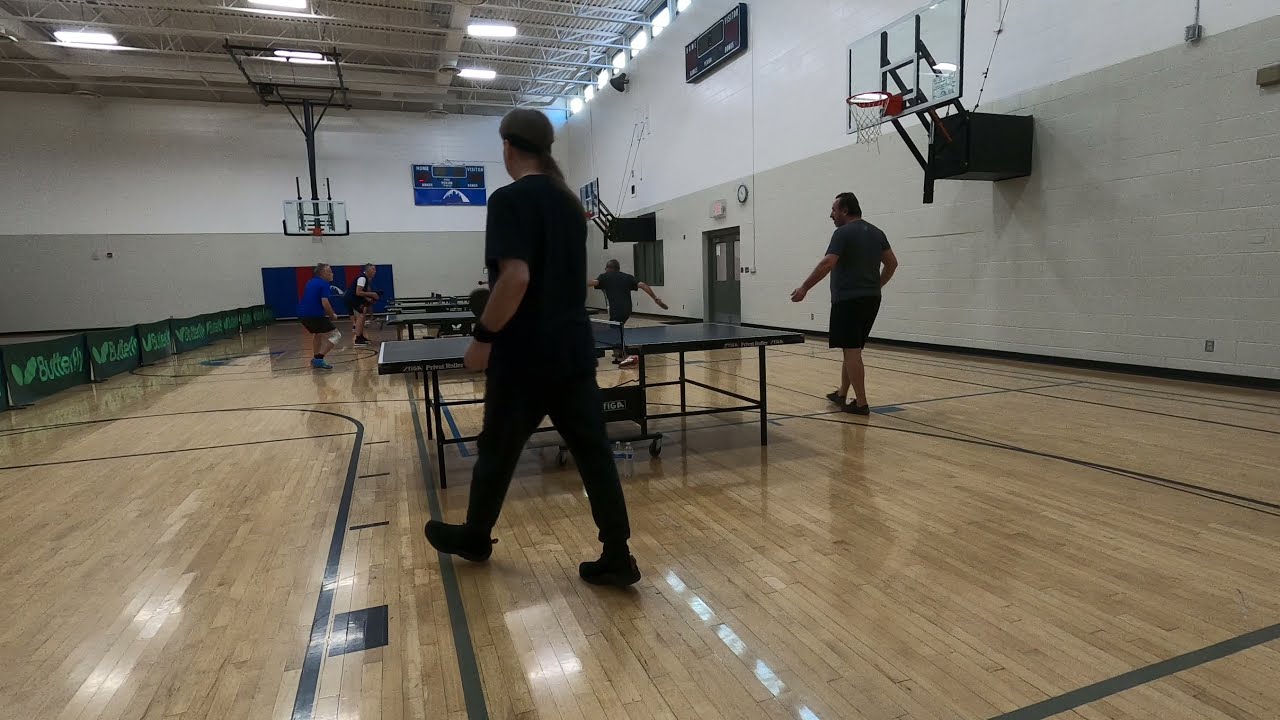The photograph captures a two-story tall gymnasium with a polished, brown wooden floor marked by green basketball court lines. The expansive space, appearing to be a recreation center, houses several parallel ping pong tables. Two of these tables, located closer to the viewer, are unoccupied, while in the background, two tables are actively hosting games. Players can be seen, including one in a bright blue shirt and others in darker attire. Two men with their backs to the camera, both dressed in black, are walking away. One of these men, most clearly visible, has long hair tied in a ponytail, and wears black pants, a short sleeve black shirt, and black sneakers, heading towards the players. The gym's dark gray lower walls and light gray upper walls are accentuated by multiple basketball backboards and scoreboards. Additional green barriers line the sides, separating the ping pong tables. The gym is well-lit by overhead lights suspended from the steel roof.